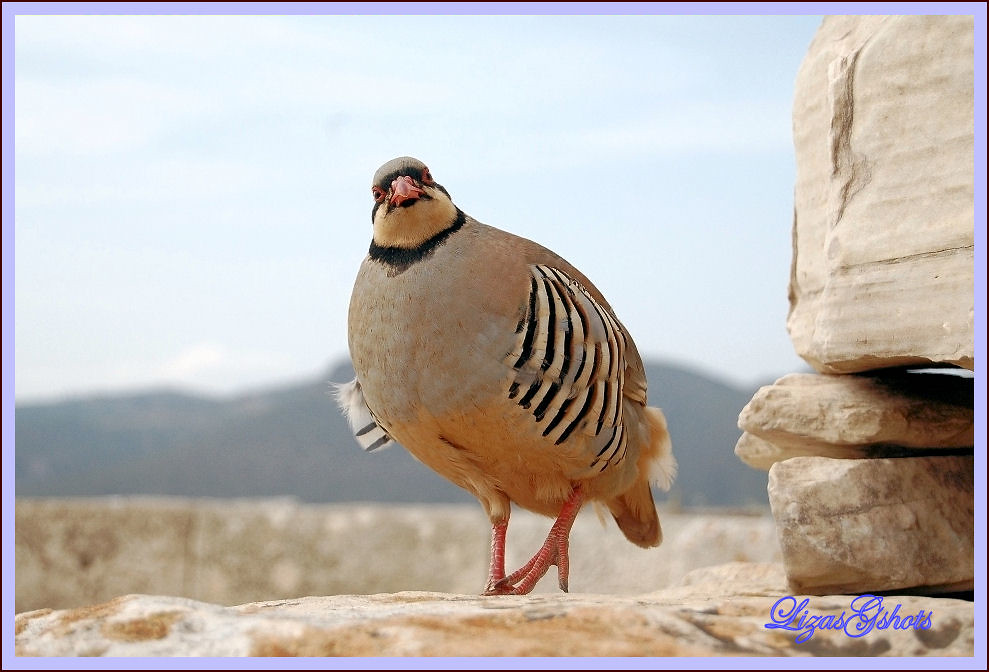This digital photograph captures a gray partridge-like bird, possibly a quail, standing on rugged, limestone-like rocks. The bird, bathed in daylight from the upper left, is looking directly at the camera with its head turned slightly to the left. It features distinctive black and white stripe patterns on its wings, a dark ring around its neck, orange eyes, and reddish feet. The scene is framed by a purple trim with a cursive signature at the bottom reading "Lasis G-Shots." In the blurred background are green mountains and sparse cloud cover, evoking a location that could be in the American Southwest, such as Utah. The overall color palette includes gray, brown, green, blue, white, and touches of purple.